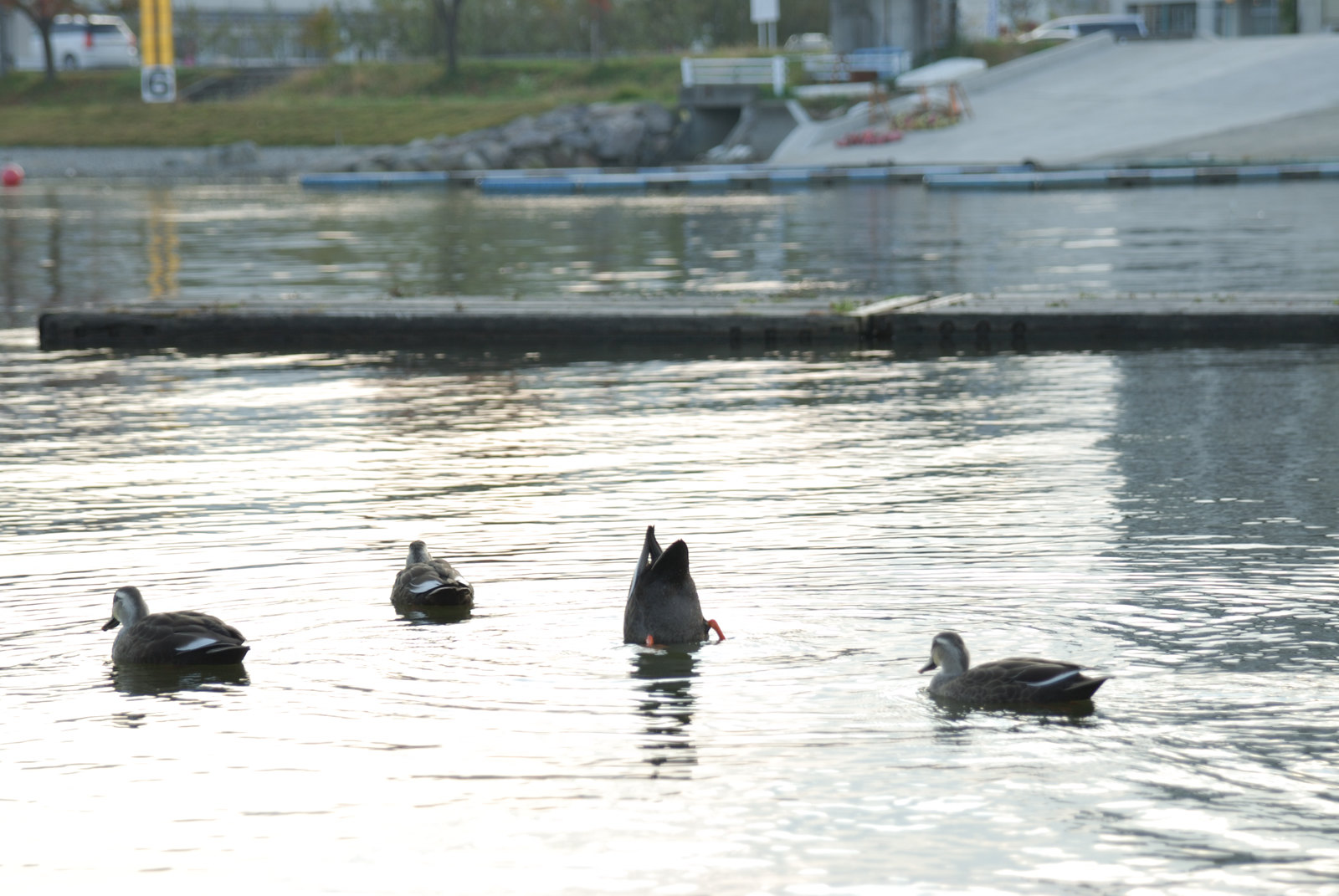In this vibrant, sunny day photograph, four ducks gracefully swim in a man-made body of water, creating delicate ripples. The duck in the center raises its body, revealing its claws, while another dips its head into the water, leaving only its tail and orange legs visible. The ducks, displaying a blend of gray and white feathers, are the focal point in front of a metallic pier that juts into the water. Further back is a paved driveway or concrete ramp leading up to a green landscape. In this area, two yellow poles marked with the number six stand out, and a white van drives along a distant road. A bright red ball floats in the water, possibly marking a boundary, while blue and black floating bars create additional interest. The whole scene is bathed in sunlight, casting a glow on the water's surface.